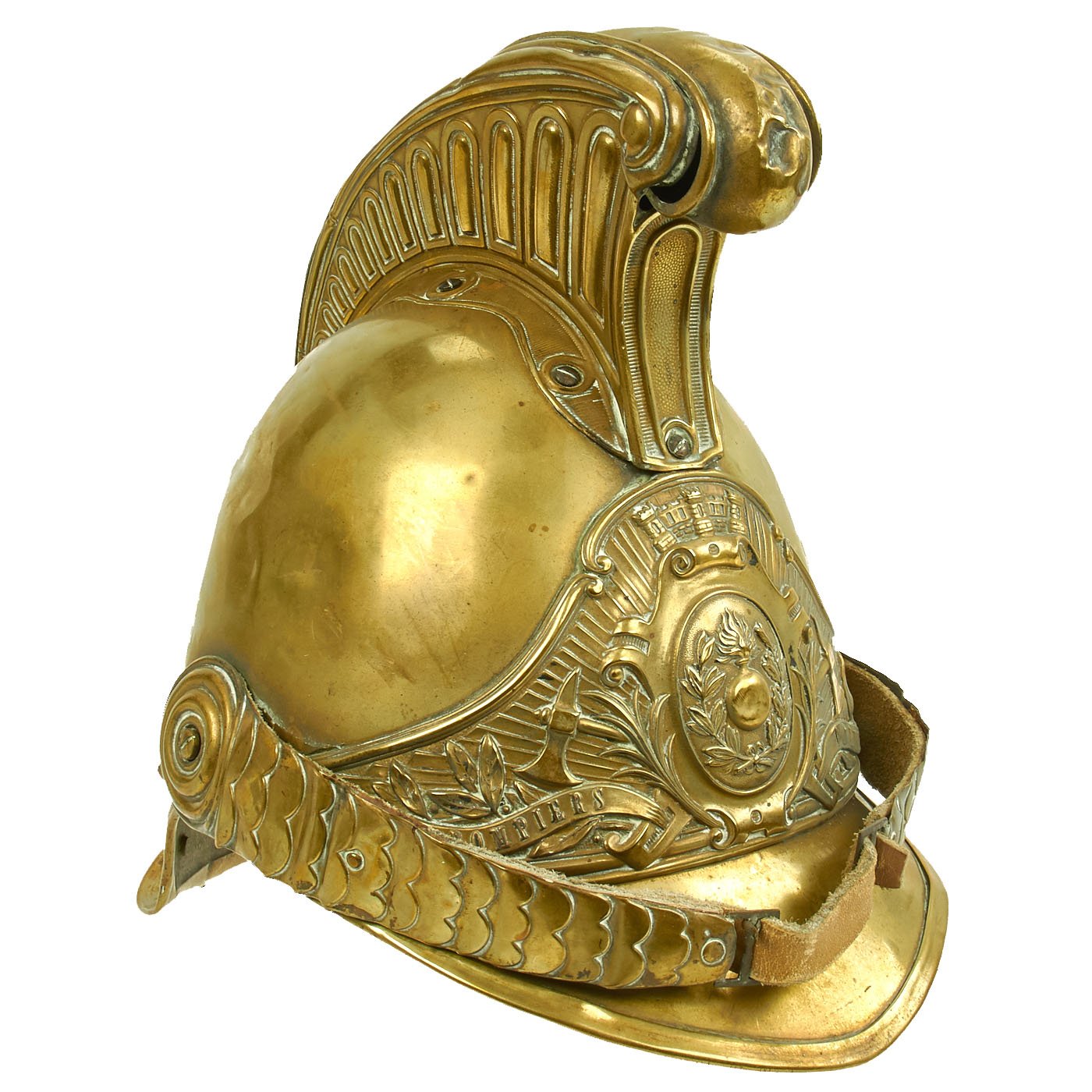This image showcases a highly detailed gold or bronze-colored helmet, evocative of both historical European military styles and formal ceremonial wear. The helmet is positioned at a three-quarter view angle against a plain white background, emphasizing its polished and reflective surface. The main structure resembles a firefighter's helmet with a distinctive, upward-curving crest, reminiscent of a Roman centurion's plume.

The front of the helmet features a built-in visor with a heavily engraved motif of leaves and a circular design with flower etchings. Above this visor, there's a raised chin strap folded up, secured by a light brown leather piece. This strap is intricately designed with engravings and would typically be unlatched to go around the wearer's chin.

On the back, the helmet has a strap that extends to a hinge on the left side, accompanied by layered detailing and a swivel mechanism for adjustment. The crown and sides of the helmet are smooth and highly polished, capturing light in a way that gives off a glowing, yellow burst effect. The top of the helmet features an elaborate upward crest that tapers to a ball-like end, further adorned with vertical scrolls and ornate patterns.

Overall, the helmet is an exquisite blend of functional design and artistic craftsmanship, likely belonging to a ceremonial guard or officer from a historical period.